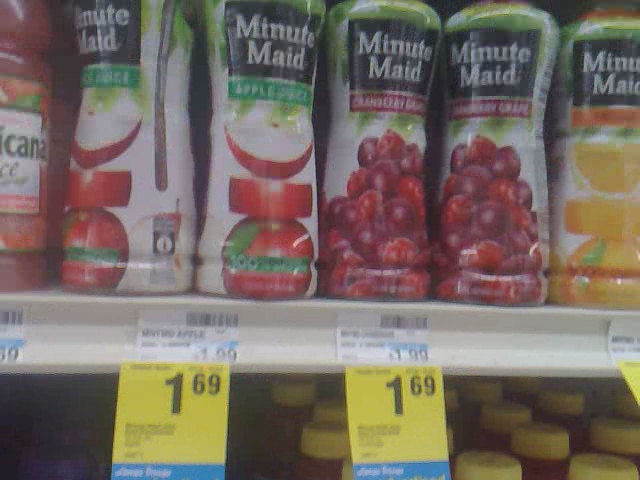This snapshot captures a vibrant grocery aisle brimming with an array of Minute Maid juice bottles adorned with different flavor labels. At the top of the image, a sale sign indicates the reduction in price from $1.99 to $1.69. Dominating the scene, the Minute Maid brand is instantly recognizable, with each bottle featuring distinct fruit imagery. 

On the left, a large container of Tropicana juice stands out in the corner, contrasting with the predominantly Minute Maid-filled shelves. The first bottle in the series showcases crisp, sliced apples, unmistakably signaling apple juice. Next in line, a bottle adorned with cranberries points to cranberry juice. Following this, a bottle with a mix of peaches or oranges, possibly mangoes given the orange hue, catches the eye. Another bottle displays enticing raspberries, promising a refreshing drink.

At the bottom of the shelves, numerous bottles with yellow tops and a variety of juices, including a reddish one, are visible, adding to the rich assortment. The overall impression is one of a well-stocked juice aisle with excellent deals available, tempting shoppers with both variety and value.